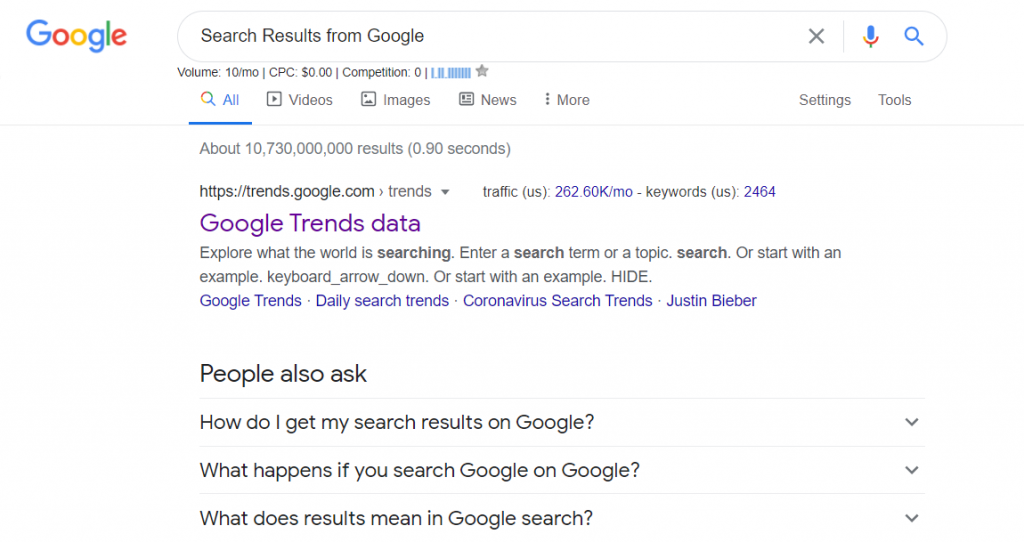The image is a screenshot of the Google search results page. In the top left corner, the Google logo is displayed, with each letter in a different color: the "G" is blue, the first "O" is red, the second "O" is yellow, the "G" is blue again, the "L" is green, and the "E" is red.

Below the logo, there's a text line that reads "Search results from Google," followed by 'X', a microphone icon, and a magnifying glass icon. On the page, there is a section displaying search metric details: "Volume, tens/mo," "CPC $0," and "Competition 0." This section includes indicators like lines and a star symbol.

Underneath, a navigation bar lists options with "All" highlighted in blue with a blue underline. The bar also includes a magnifying glass icon and a rainbow, along with other tabs labeled "Videos," "Images," "News," and "More." 

To the right, links for "Settings" and "Tools" are present. Further down the page, the text reads: "About 10,730,000 results in 0.90 seconds."

Additionally, there's a "People also ask" section with several dropdown questions:
- "How do I get my search results on Google?"
- "What happens if you search Google on Google?"
- "What does 'results' mean in Google search?"

The screenshot illustrates typical elements of a Google search interface, complete with search options, metric details, and related questions displayed on the results page.